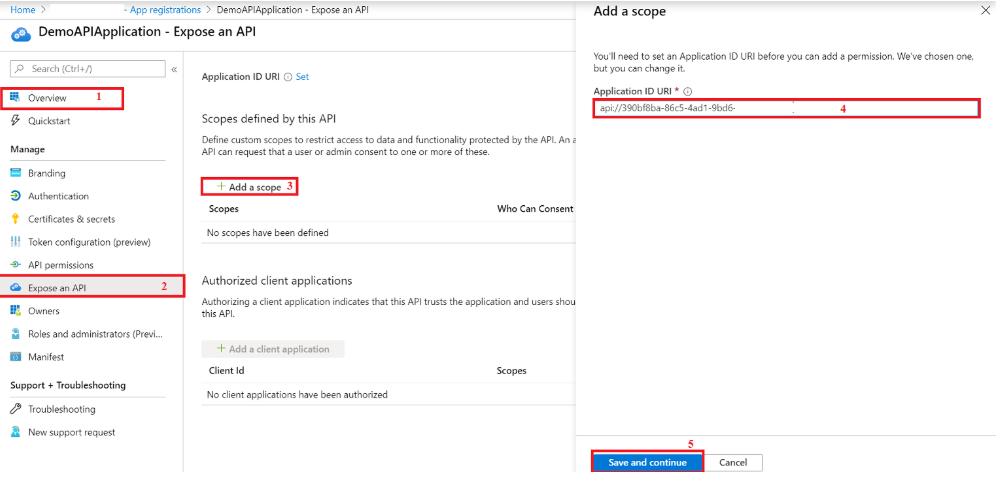This image appears to be a detailed demonstration for configuring an API application within a software interface. At the top, navigation options are visible, including "Home," "App Registrations," "Demo App API Application," and "Expose an API," with "Home" and "App Registrations" text highlighted in blue. A blue cloud icon featuring two circular elements is also present for visual emphasis. 

In the upper section, titled "Demo API Application – Expose an API," a search box adorned with a magnifying glass icon provides the capability for quick searches. The shortcut "[Ctrl + /]" is indicated beside it. An expandable menu, marked by double left-pointing arrows, precedes an overview section that contains a chart illustrated with three small squares and a magnifying glass icon, labeled "Overview" with a red notification badge indicating attention is required.

The walkthrough is annotated with red boxes numerically ordered to show the steps. Step 1 features a red box around "Overview." Below, a "Quick Start" section is identified by a lightning bolt icon. Under the "Manage" section, various subcategories, such as "Branding," "Authentication," "Certificates & Secrets," "Token Configuration Preview," "API Permissions," and others, are accompanied by respective icons.

Step 2, boxed in red, is around "Expose an API," including sub-options for "Owners," "Roles and administrators," "Manifest," "Support and troubleshooting," and more. The application ID URL is circled with an information icon for further details. A critical explanatory box states, "Scopes defined by this API," instructing users on defining custom scopes to control access, with the bolded question "Who can consent?" highlighted.

In Step 3, identified by another red box, users are instructed to "Add a scope," marked by a green plus sign. It's noted that "No scopes have been defined." Further down, the section "Authorized client applications," which includes a grayed-out button labeled "Add a client application," specifies the absence of authorized client applications and re-emphasizes the scopes and permissions.

Step 4 highlights the "Application ID URL" with required input fields and features a circuited information icon. The value provided is "API://390BF8BA-86C5-481-9BD6," encased in a numbered red rectangle.

Finally, Step 5 underscores the "Save and Continue" button, blue with white text, and the adjacent "Cancel" button, white with black text, completing the configuration process.

This annotated screenshot vividly outlines the multi-step process to add and expose an API within the application, guiding users through an intuitive, step-by-step interface configuration.